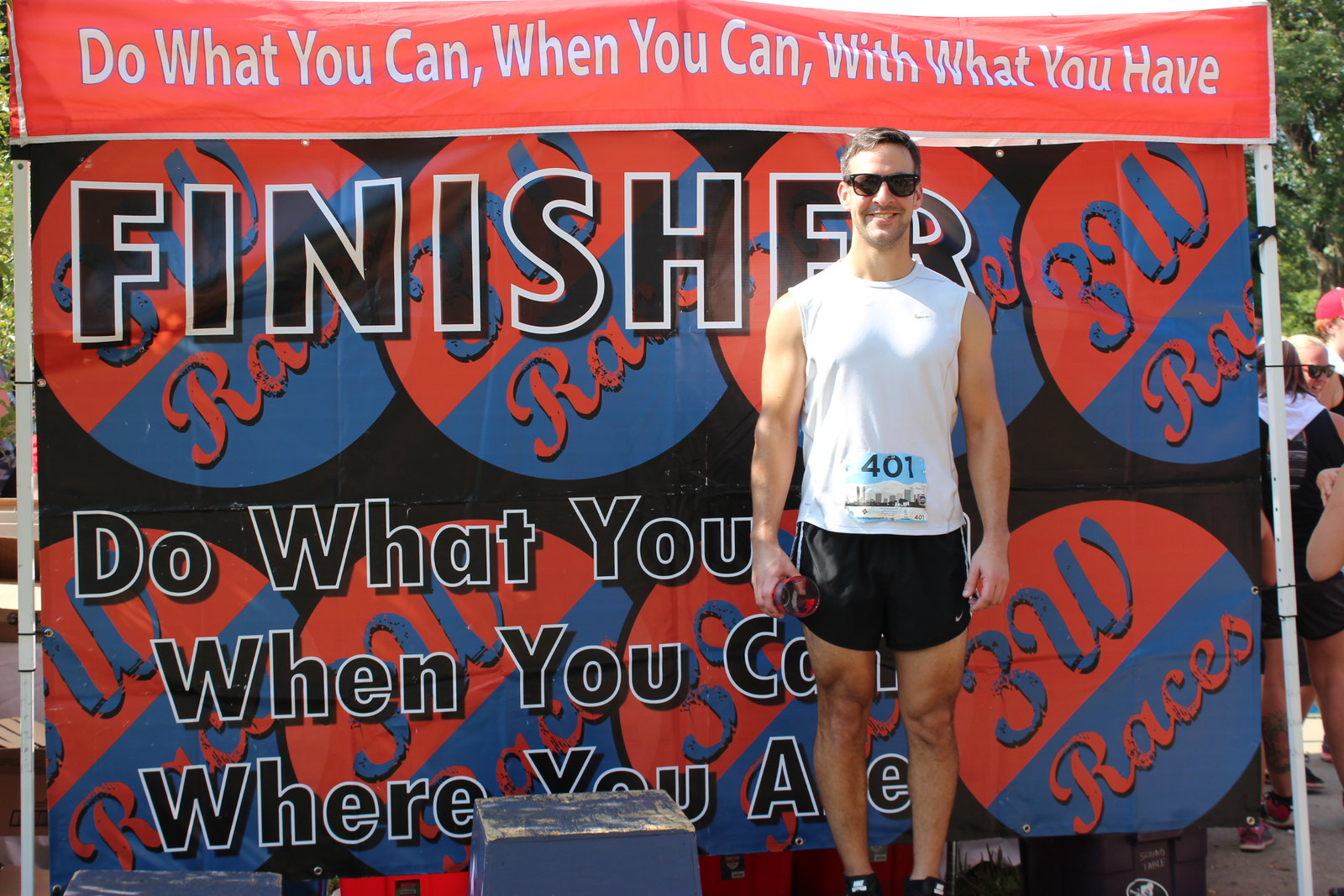The image depicts a very fit white male, appearing to be in his late 30s or early 40s, who has just finished a competitive run. He is wearing sunglasses, a white sleeveless runner's shirt with the number 401, and black shorts that reach the middle of his thighs. He stands on a winner's platform, likely in the third position, holding a cup in his hand and smiling. Behind him is a large tarpaulin banner supported by white poles, featuring a red top section with white text that reads, "Do what you can, when you can, with what you have." The banner also includes circles with the letters "3W races" on them, indicating the charitable run he participated in. The word "Finisher" is prominently displayed in white-outlined black text. Some people are visible in the background, but their activities are unclear. This man is likely posing for a photograph to commemorate his achievement and share with his family.